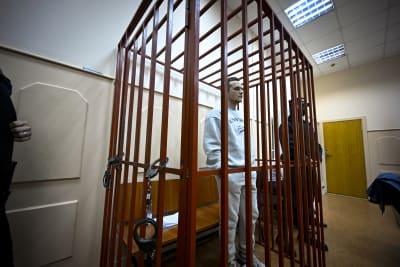The photograph depicts a young Caucasian man standing calmly inside a makeshift, portable red cage, which resembles a small cell situated within a larger room, likely a courtroom or office environment. The man, dressed in a light gray sweater and sweatpants, stands with his hands in his pockets, facing forward. Inside the cage, which has bars painted reddish-orange, there is a wooden bench with a small stack of papers on it. Handcuffs are attached to the bars on the left side of the cell, though the man himself is not restrained by them. Two guards dressed in blue flank the cage, one of whom appears to be wearing a mask. The room surrounding the cage has paneled walls and a wooden beige door, contributing to an older, office-like atmosphere.